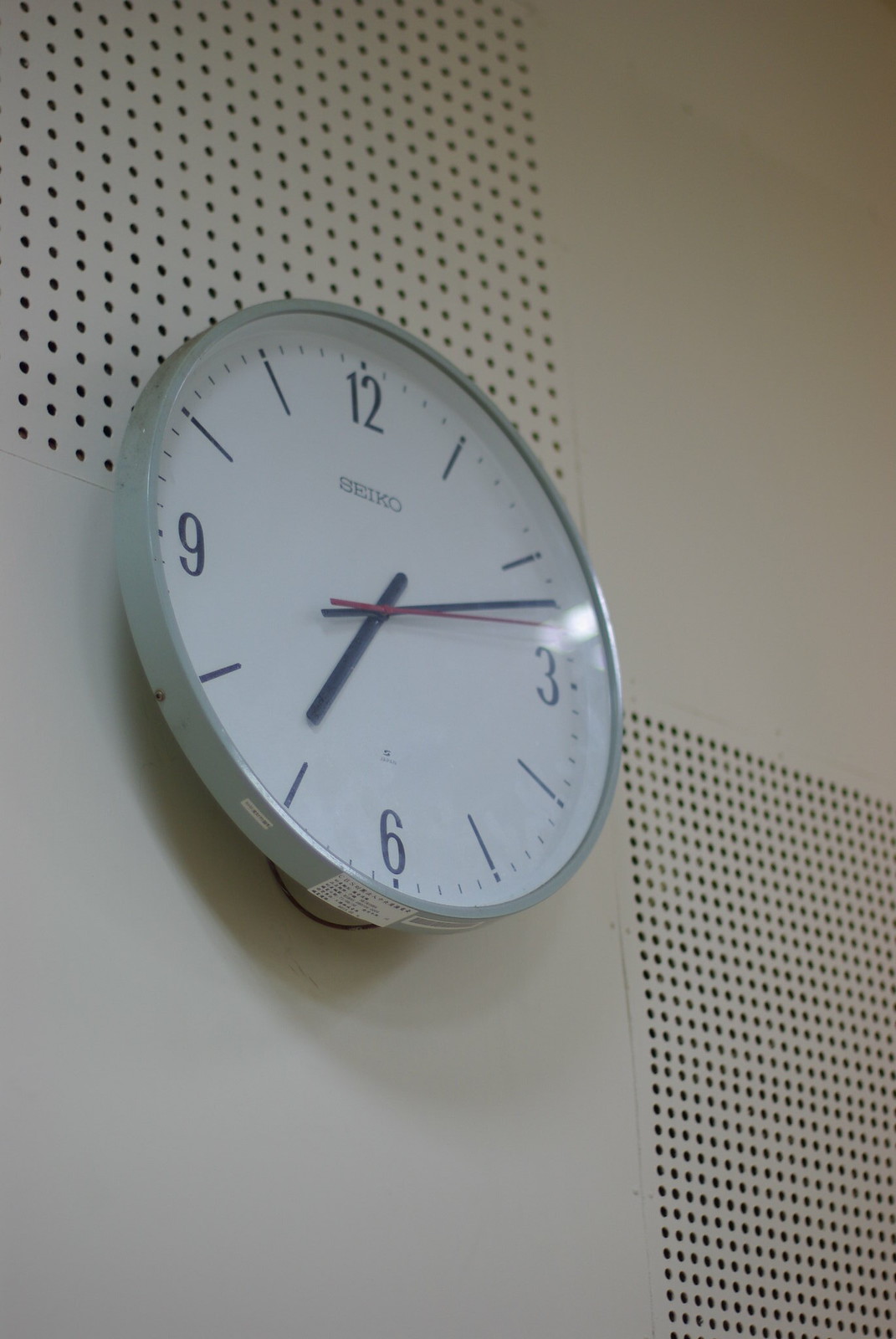This indoor color photograph captures a wall-mounted clock from a low-angle perspective, tilted upwards at approximately a 45-degree angle and slightly diagonal to the left. As a result, the nine on the clock face is prominently closer to the viewer. The clock, featuring a minute, hour, and second hand, shows the time as 12 minutes past seven. The hour and minute hands are black, while the second hand is red, positioned just one increment past the minute hand. 

Notably, the clock is mounted away from the wall, revealing a circular shape at the bottom that seems to be a wire, suggesting it is electrically powered rather than battery-operated. A thin black wire droops down in a slight arc behind it. Additionally, there is an unreadable sticker with writing on it located at the bottom of the clock. The clock's rim, encircling its circumference, is colored in a light greenish-grey hue.